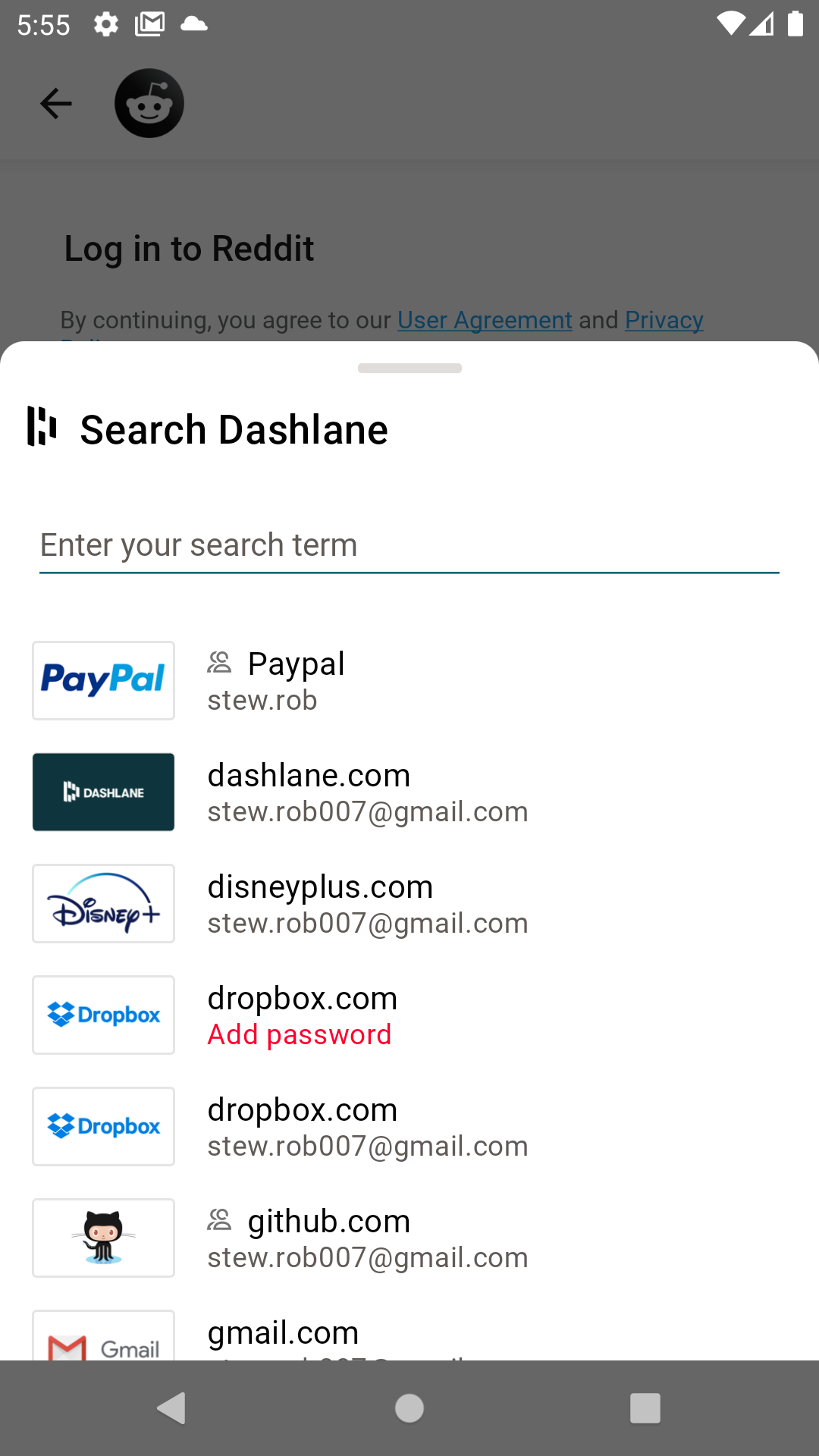In this image, we see a device screen. At the top left, the time is displayed as "5:55." Moving to the right, there's a settings icon, followed by an email icon, and then a cloud icon. On the top right are three additional icons: a cellular signal indicator, a Wi-Fi symbol, and a battery icon.

Below this top bar, towards the left, there is a black arrow pointing to the left. Next to this arrow is the Reddit logo. Below the logo, text reads: "Login to Reddit. By continuing, you agree to our User Agreement and Privacy." 

Further down, there is a search bar that states, "Search Dashlane" with a placeholder text "Enter your search term." The search bar is underlined by a dark green line stretching across from left to right.

Beneath the search bar, there appears to be a series of tabbed sections. The top tab is labeled "PayPal," followed by another tab labeled "stu rub," and the last visible tab reads "dashlane.com."